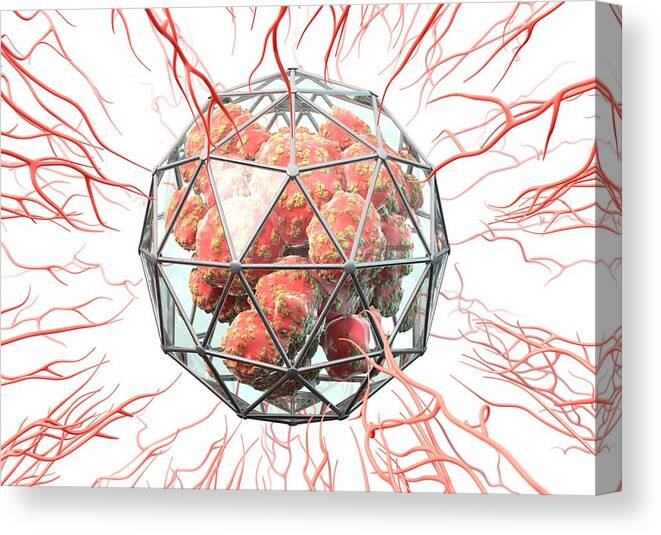The image is a three-dimensional canvas painting, depicting an intricate and captivating scene. At the center of the artwork is a glass sphere, shaped like a decahedron with numerous triangular facets held together by thin silver metal strips. Inside this glass structure are brown, ball-like clusters that have a mold-like appearance with various lighter gray specks and spots. Surrounding the glass sphere, countless red blood vessels extend outward, creating a complex network that seems to converge towards the central barrier. Additionally, branches or tree roots emerge from different sides of the canvas; they are brown at the top left and center, transitioning to a white or cream color as they wind their way in various shapes and directions. This richly detailed painting, photographed at an angle, accentuates its three-dimensional quality, making it an intriguing piece likely intended for household decor.